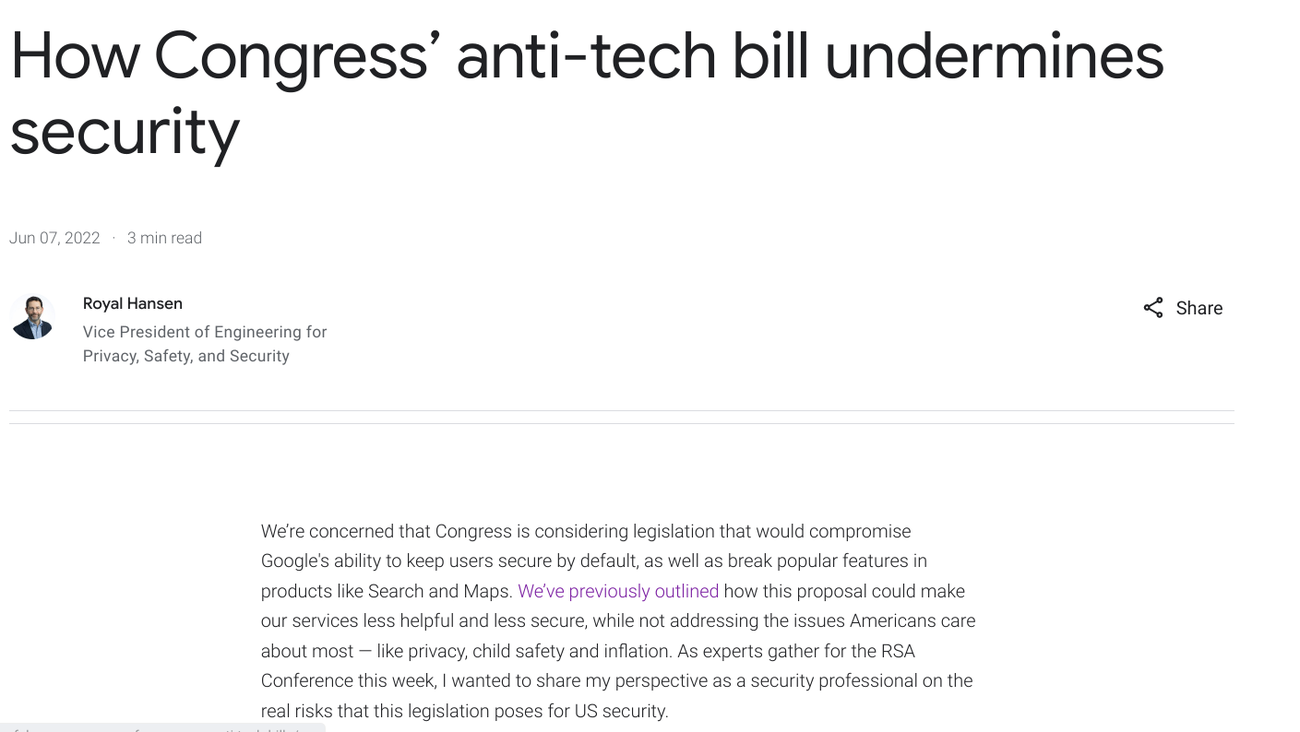**Title:** How Congress's Anti-Tech Bill Undermines Security

**Details:** The image features a white background with text prominently displayed on the left. At the top in black text, it reads: "How Congress's Anti-Tech Bill Undermines Security." Below, it states that the article was posted on June 7, 2022, and it mentions that it is a three-minute read. The author is identified in black text as Roy Johansson, Vice President of Energy and Neighborhood for Privacy, Safety, and Security. 

Two horizontal gray lines separate the title and the main content. The body of the text is in black and starts with a short paragraph expressing concern about Congress considering legislation that could compromise Google's default security measures. It notes the potential negative impact on popular features like Search and Maps. Highlights in purple emphasize the message, stating, "we previously outlined," and reverting to black to explain how the proposal could make Google's services less helpful and secure. 

The text criticizes the bill for not addressing key issues such as privacy, child safety, and inflation, which are top concerns for Americans. A section in all capital letters mentions an upcoming "CONFERENCE" this week, where experts will gather. The author, identified as a security professional, wishes to share his perspective on the real risks that the legislation poses for U.S. security.